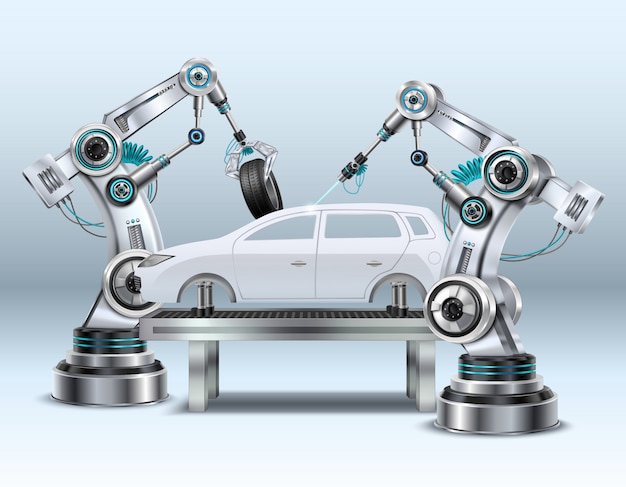The image depicts a computer-generated scene of a white, four-door sports sedan in the process of being constructed by automated factory machines. The car, streamlined and wheel-less, is elevated on a silver metal platform supported by four small pillars. In the foreground, two advanced robotic arms are engaged in different tasks. The mechanical arm on the left features a grasping claw that is maneuvering a tire towards the car, while the arm on the right appears to be emitting a laser beam at the vehicle's body, possibly performing a welding operation. Both robotic arms are made of stainless steel with blue wiring and are equipped with various tools and pulley mechanisms. The background is a silvery light blue, giving the entire scene a futuristic, AI-driven ambiance.